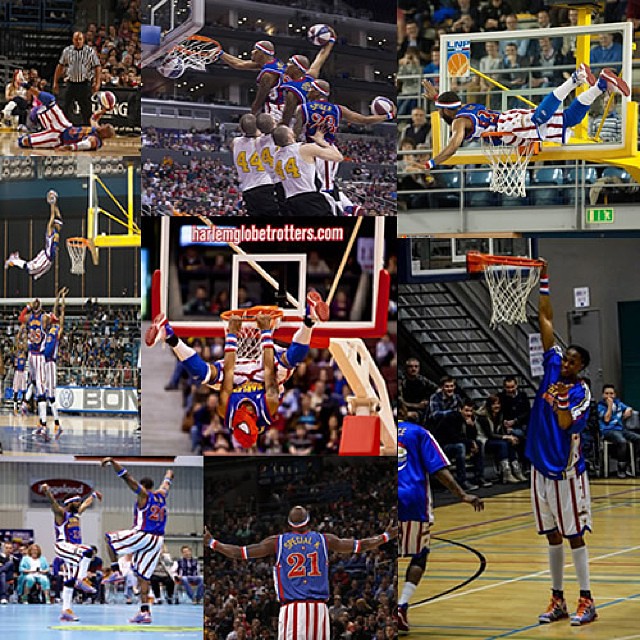The image is a perfectly square collage of nine different photographs featuring the Harlem Globetrotters in their iconic blue jerseys and red-and-white striped shorts adorned with stars. The photographs are thoughtfully arranged with four on the left, three in the center, and one on the right. In the middle of the collage, a player hangs upside down from a basketball hoop wearing a Spider-Man face mask, emphasizing the playful and entertaining nature of their performance. Surrounding this central image are various captivating shots: 

- Top left: A player is on the ground with a basketball while a referee approaches him.
- Upper right: A player impressively lies across the basketball rim next to the backboard.
- Lower left: Two players are seen doing a Karate Kid-like stork pose.
- Middle center: A player stands with arms raised, exuding confidence.
- Middle left: A player flies through the air in the middle of a dunk.
- Bottom right: A player touches the basketball rim effortlessly without standing on his toes, and another image shows a player perched on top of the hoop. 

Each photograph eloquently captures the dynamic and amusing stunts for which the Harlem Globetrotters are renowned. The text "HarlemGlobetrotters.com" is prominently displayed in white letters with a red border at the center, drawing attention to the team's official website.